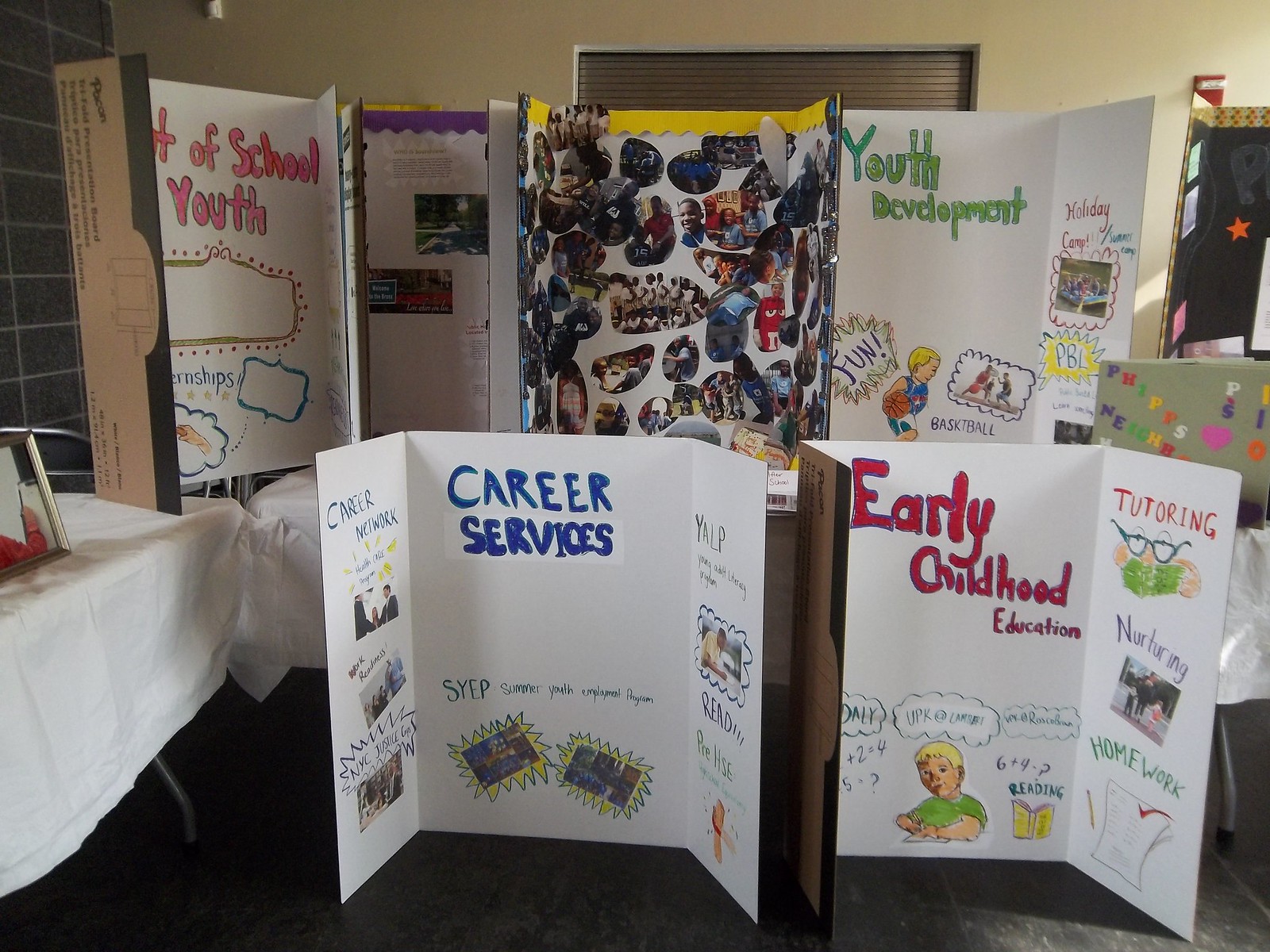The image displays a series of detailed cardboard poster boards, presumably for a school project or event, arranged on tables draped with white tablecloths. At the center, a prominent collage of numerous photographs is visible, portraying students engaged in various activities. Around this central poster, six distinct boards cover diverse educational topics: youth development is highlighted in green, showcasing pictures of kids participating in sports; early childhood education stands out in red, featuring student drawings and the words "tutoring," "nurturing," and "homework"; career services is marked in blue and includes photographs and text. Another poster focuses on school youth, though full details remain partially hidden. The scene is set against a background with peach-colored walls, two visible windows, and a gray floor, enhancing the vibrant educational atmosphere.